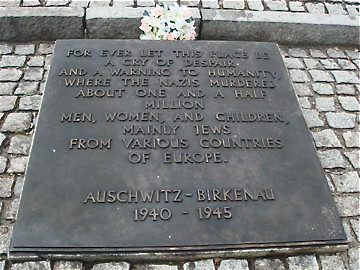The image depicts a solemn Holocaust memorial consisting of a large, dark-colored stone tablet mounted on a wall of gray and white bricks. The tablet bears a deeply etched inscription that reads: "Forever let this place be a cry of despair and a warning to humanity where the Nazis murdered about 1.5 million men, women, and children, mainly Jews, from various countries of Europe." Below this poignant message, the tablet is marked with "Auschwitz-Birkenau, 1940-1945." In front of the tablet, on the ground next to a curb, lies a bouquet of pink and white flowers, adding a touch of color to the otherwise somber scene. The material of the tablet appears to be bronze, suggested by its dark hue and the lack of rust spots, adding a timeless quality to the memorial. The overcast, gray day further accentuates the somber and reflective atmosphere.